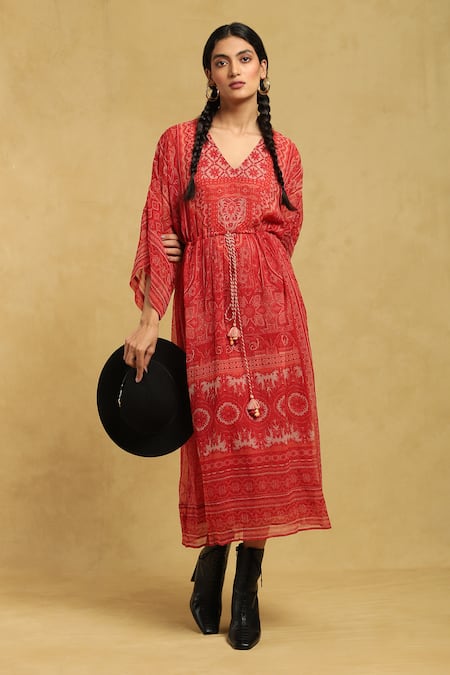The image showcases a striking, young woman standing confidently in what appears to be a professional photography studio with a tan backdrop. The woman, reminiscent of Salma Hayek, has deep black hair styled into two long braids that fall elegantly over her chest. She is dressed in a vibrant, free-flowing red dress adorned with intricate patterns, possibly Native American-inspired, and accentuated with three-quarter sleeves and a V-neckline. The dress features a chain detail that adds a touch of modernity to its traditional design.

Her attire is complemented by black high-heeled boots that reach to mid-ankle, enhancing her poised yet relaxed stance. She holds a black hat from the top in her right hand while her left hand is positioned behind her back, clutching her elbow, adding to her statuesque posture. The woman's accessories include notable gold hoop earrings, which glint against her minimal makeup, highlighting her natural beauty.

The overall setting, with its bold yet neutral tones of orange, red, and taupe, further emphasizes the model's striking presence against the tan floor and background. She gazes directly into the camera, exuding an air of confidence and elegance, quintessential for a fashion model presenting a blend of traditional and contemporary attire.